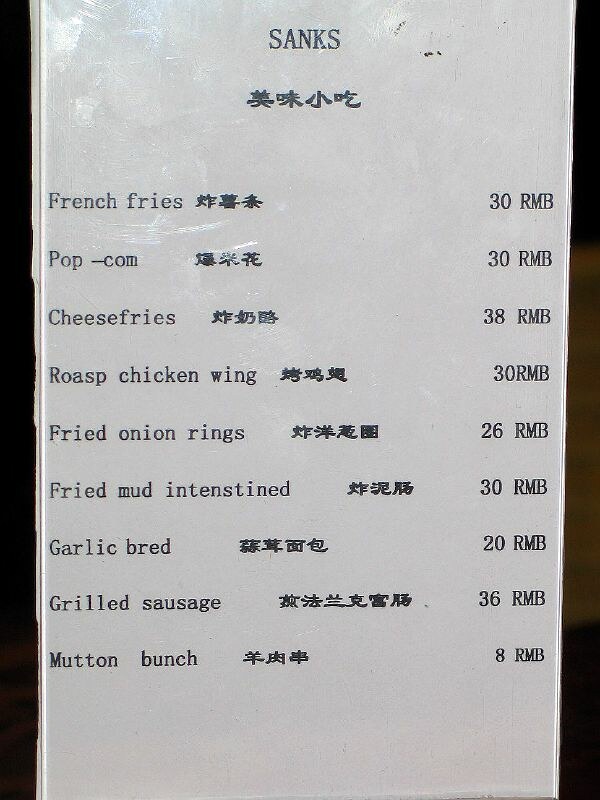The image shows a laminated restaurant menu presented in both English and Mandarin. The menu stands upright and prominently displays "SANKS" in large black capital letters at the top, with its Mandarin equivalent directly underneath. Each food item is listed with its corresponding name in both languages, along with its price in RMB (Chinese Yuan). 

The listed items and their prices are as follows:
- French Fries: 30 RMB
- Popcorn: 30 RMB
- Cheese Fries: 38 RMB
- Roast Chicken Wings: 30 RMB
- Fried Onion Rings: 26 RMB
- Fried Intestines: 30 RMB
- Garlic Bread (spelled as "Bred"): 20 RMB
- Grilled Sausage: 36 RMB
- Mutton Butt: 8 RMB

The menu reflects a diverse selection of items, each accompanied by its price in the local currency, which the creator believes to be Chinese Yuan (RMB).